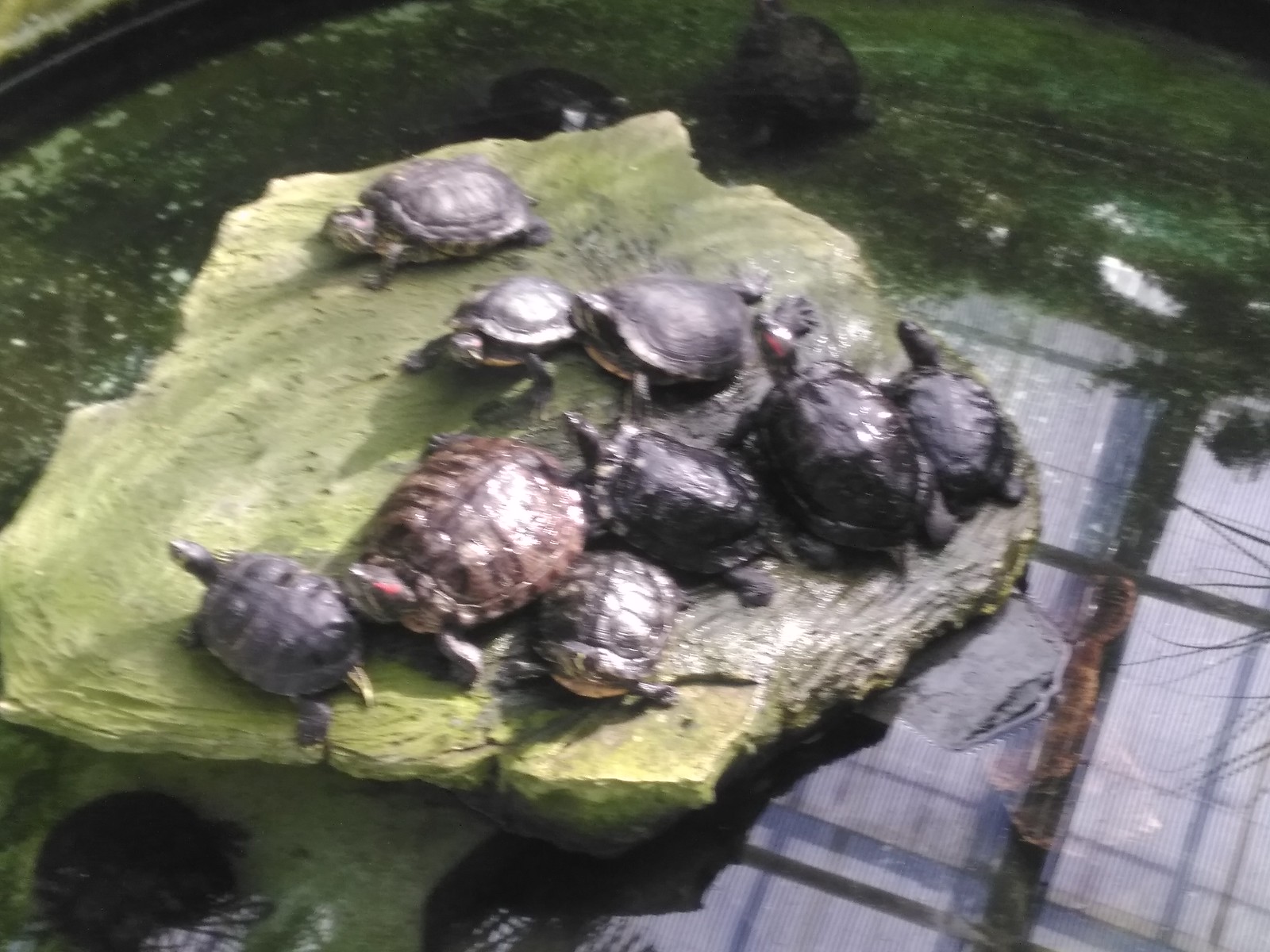A blurry photograph captures a small pond, likely in a zoo or enclosure, encircled by what appears to be a plastic rim. The water is a dark, algae-filled green, reflecting a plaid pattern possibly from a piece of cloth with a white background and blue and black checks. Rising from the pond is a large green rock. This rock is the focal point for a bustling collection of turtles, most of which are dark gray or black with similar-sized shells. Positioned strategically on the rock, some turtles are sunning themselves while others appear to be on the move. Dominating the scene are two larger turtles, one with a notably large brown shell located on the bottom left and another of comparable size on the bottom right, possibly suggesting a parental role. Surrounding them are a variety of smaller turtles, with the smallest being almost half the size of the largest. Additionally, there are approximately four turtles swimming in the dark green water. The entire scene is dotted with small plants and the surface of the water appears bubbly, adding to the natural yet contained environment.